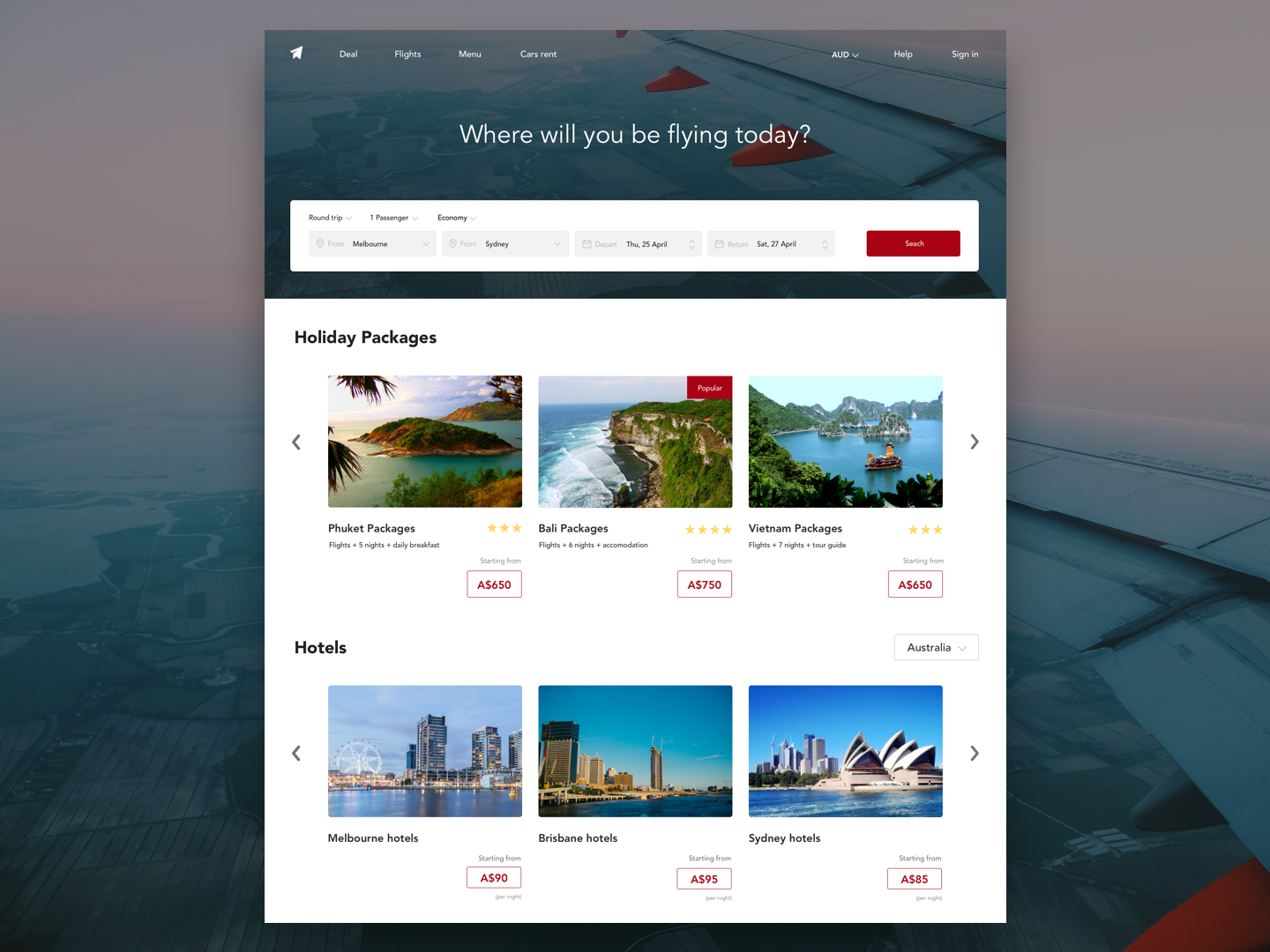A vibrant image captures a screenshot of an airline or vacation website, inviting users to explore various holiday packages and accommodations. The main focus is a prominent rectangular screen, oriented vertically, embedded within a larger background photograph taken from an airplane. The expansive sky features a serene light pink and purplish hue, while the plane's white wing extends diagonally from the right side of the photo.

At the top of the webpage, small white text offers navigational buttons. Directly beneath, in larger white text, the site prompts, "Where will you be flying today?" Below this prompt, a large white rectangular search box stands out, complete with a red search button in the bottom right corner and a variety of filter options positioned to its left.

Further down, the site showcases a row of vibrant images depicting tropical destinations, under a heading that reads “Holiday Packages” in bold black text on the top left. Directly below this section, another row is labeled “Hotels” in bold black text, featuring photos of urban landscapes with towering buildings. The entire composition effectively blends the allure of travel with the functionality of online vacation planning.